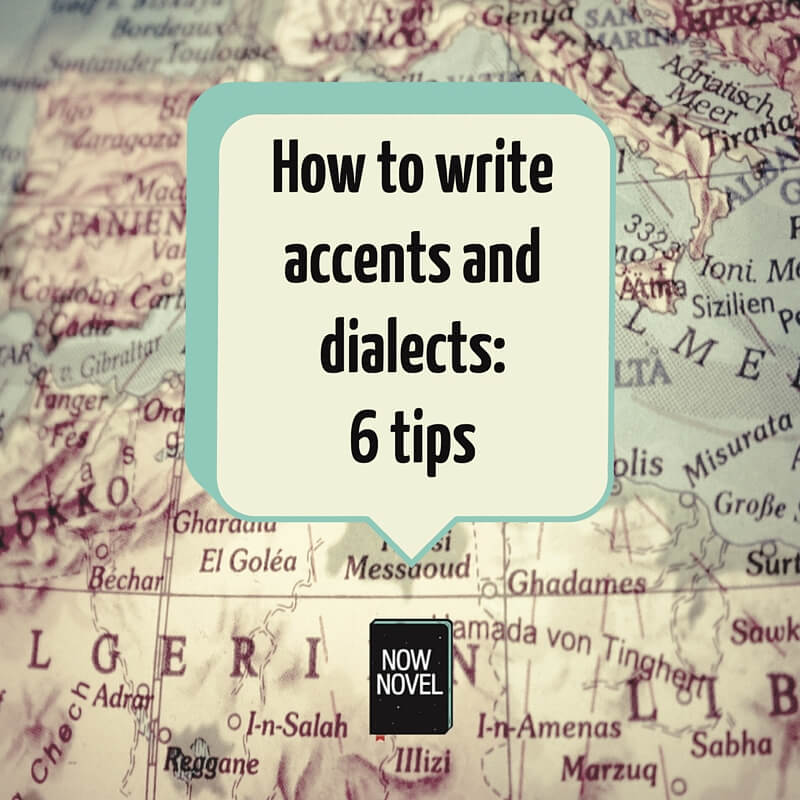The image depicts a detailed map used as the background, showcasing place names like Algeria and Liberia in brown and gray tones with black and red text. Overlaying the map, centrally positioned, is a light yellow, square text box with rounded corners and a teal shadow border. This box contains the title of a book in large, black, block letters: "How to Write Accents and Dialects: Six Tips". Below the text box extends a teal arrow-shaped protrusion pointing to a small black icon of a book labeled "Now Novel" in white text with green-tinted edges. The detailed map behind this composition adds a geographical context to the visual presentation.